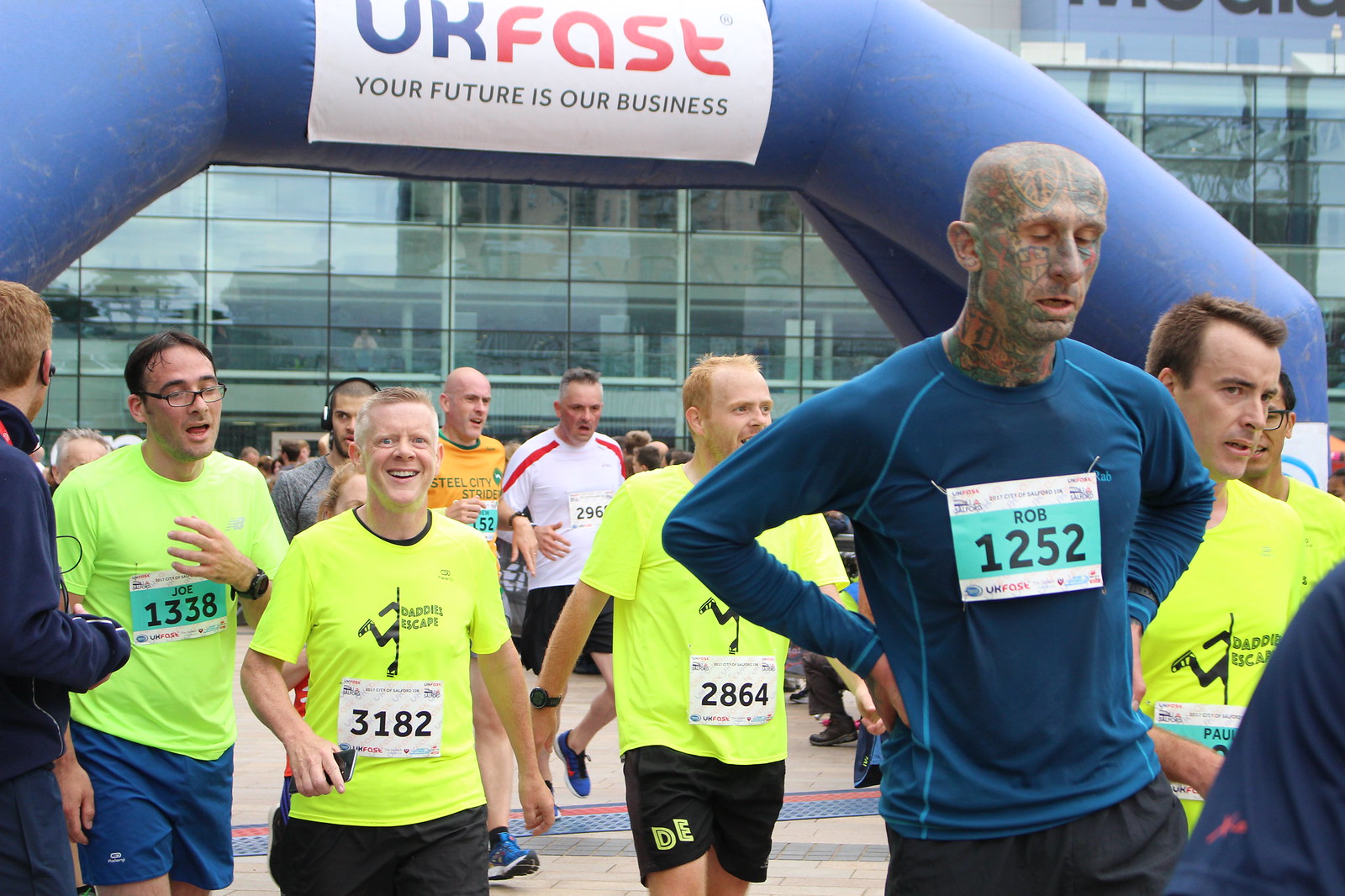This vibrant outdoor photograph captures a group of marathon runners nearing the finish line, set against the backdrop of a towering glass office building. The runners are a diverse array of individuals predominantly wearing fluorescent yellow tops, interspersed with a few in blue and white shirts. Notably, two runners sport black logos on their shirts reading "Daddy's Escape." Each participant proudly displays a numbered bib, with names such as Rob (1252) and Joe standing out. Rob, in a blue shirt adorned with head tattoos, is noticeably in the foreground. The bibs feature a mix of black, blue, and white numbers, including 1338, 3182, and 2864. An inflatable blue archway spans the background, with a bold message in blue and red letters declaring "You Are Fast," accompanied by a black subtext that reads, "Your Future Is Our Business." The scene radiates the energy and exhaustion typical of race finishers, their expressions a testament to the effort they've invested in the marathon.